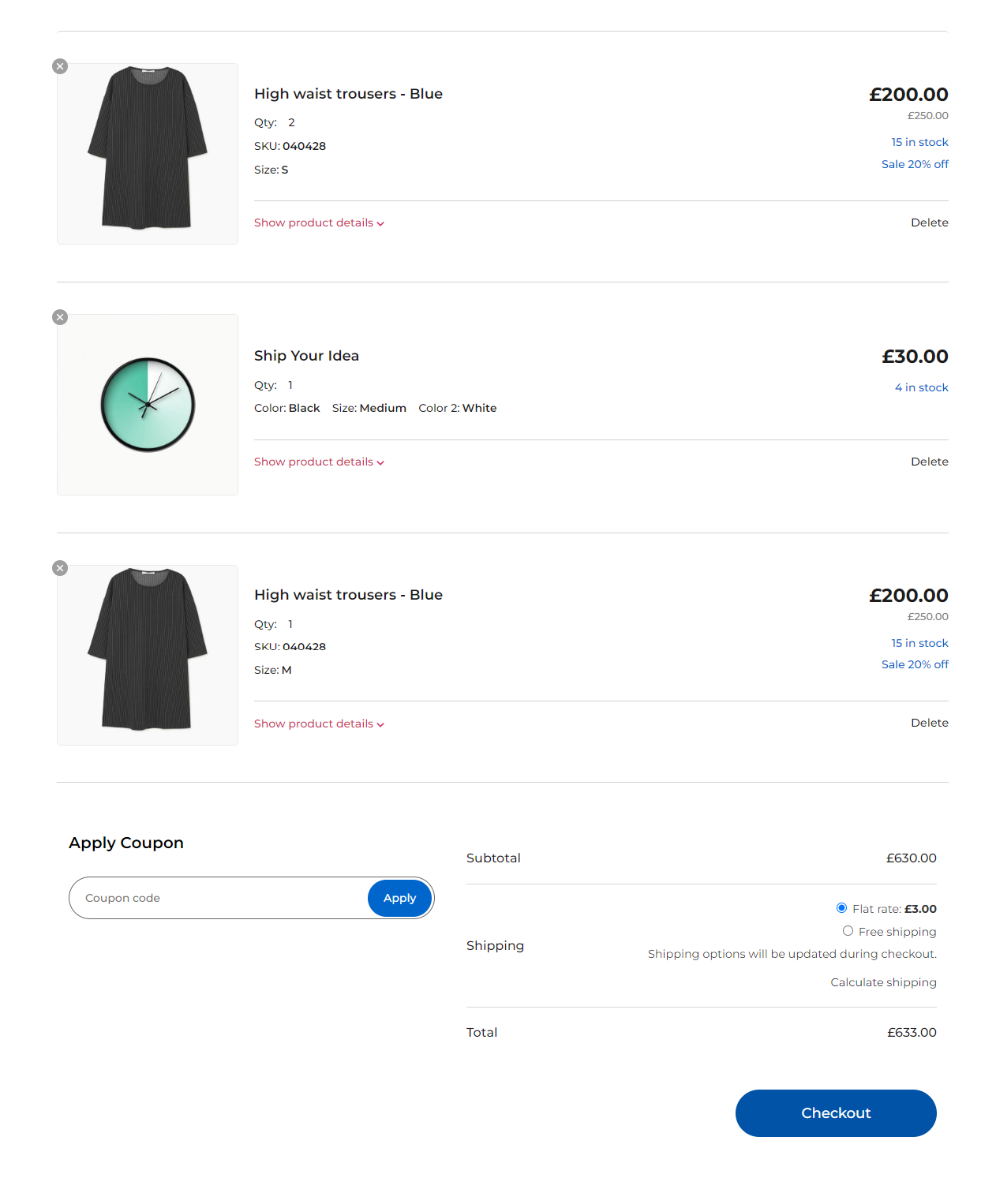A detailed, clean caption describing the photographic image of the website could be:

"The image displays a clean, white background webpage showcasing various clothing items. The first item featured is a black shirt, likely a stock image for the high-waist blue trousers described alongside it. These trousers are priced at 200 euros, with a quantity of two available. The SKU number 040428 is listed, and a red dropdown button says 'Show Product Details.' The size indicated is small. The stock information shows 15 units available in blue text, along with a 20% off sale tag and a delete option.

Following this, the next item listed is a product titled 'Ship Your Idea,' identifiable by a clock-like logo in green, black, and white. This item is priced at 30 euros, with four units in stock and a quantity of one shown. It is available in black and white, with size marked as medium. Similar to the previous item, there is a red 'Show Product Details' dropdown and a delete option.

The high-waist blue trousers are listed again, priced at 200 euros, in a medium size with a quantity of one. This entry also mistakenly displays the black shirt's stock image instead of the correct product photo."

This refined caption provides a clear and structured description of the webpage and the details of the items displayed.